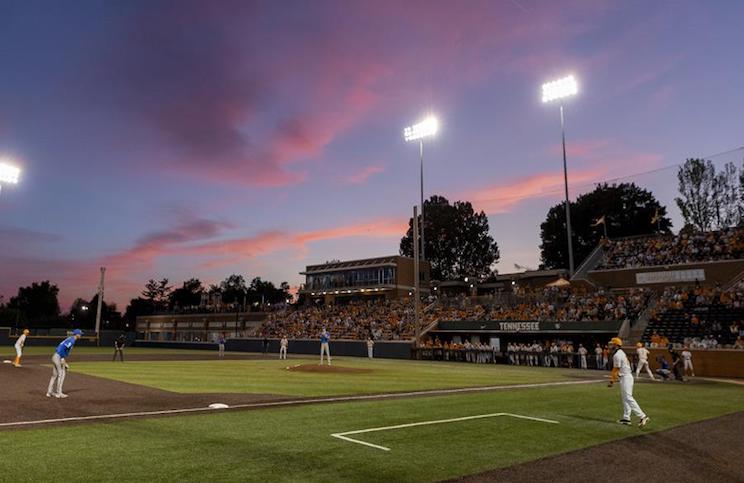This image captures an evening baseball game at a stadium, viewed from the third base side. In the foreground, the neatly mowed field features white chalk lines marking the coach’s box and bases. A coach in a white uniform with a yellow long-sleeve shirt and yellow cap stands near the third base coach's box, possibly signaling to his players. The team on defense wears blue jerseys and white or gray pants, with the pitcher standing on the mound and players positioned across the field. On offense, the team in white uniforms with yellow accents has runners on first and second bases, while the batter, wearing number one, is at the plate. In the background, a dugout with 'Tennessee' emblazoned on the header indicates that the Tennessee Volunteers are one of the teams playing. The stands have a moderate crowd, and several tall light posts illuminate the field as dusk settles in, casting a pink and blue hue across the sky. Behind the stadium, trees frame the scene, enhancing the tranquil atmosphere. The image also shows elements like the press box and players in the dugout, adding to the detailed depiction of the game in progress.